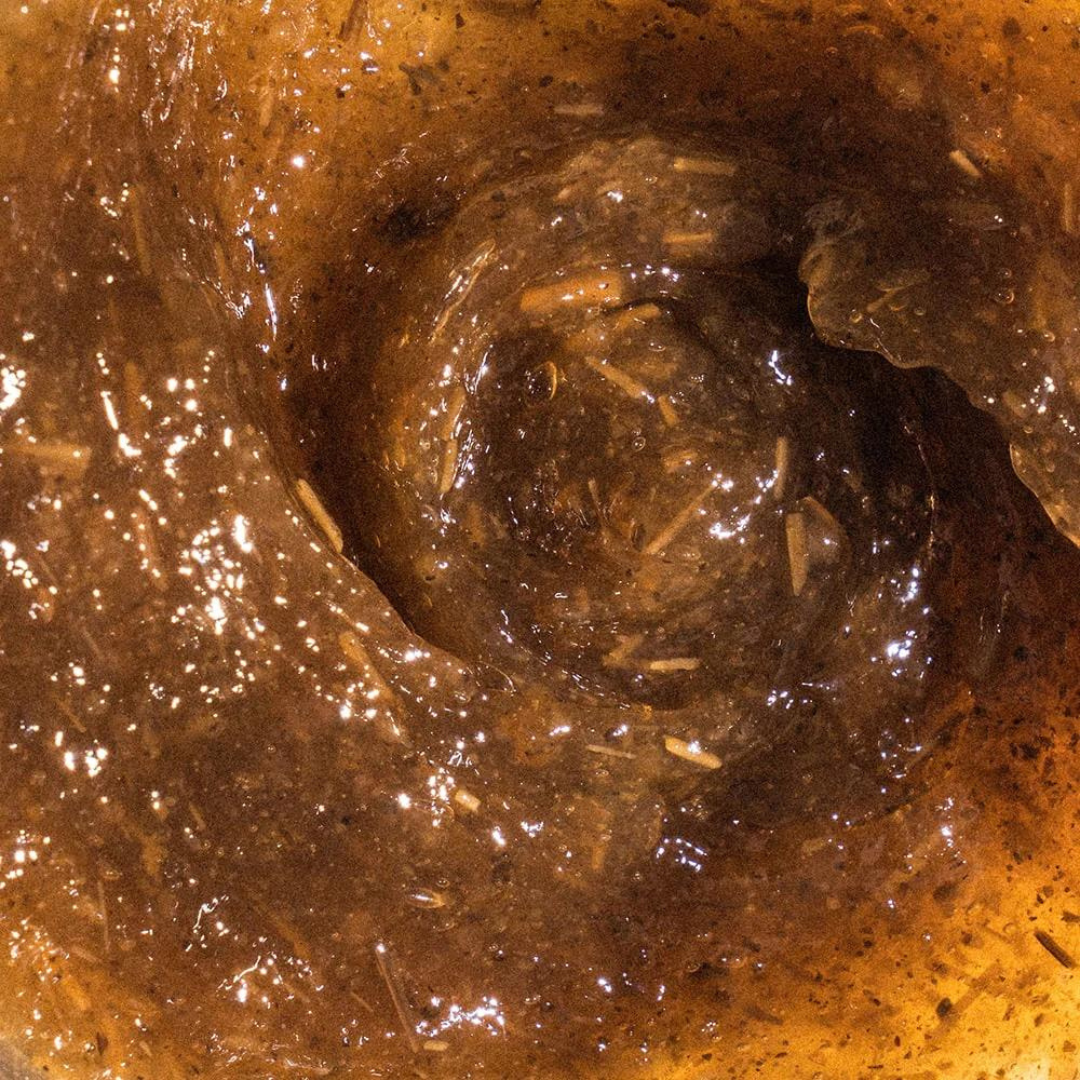This close-up photograph captures a mysterious, slimy, brown substance with a shiny texture, appearing in a spiral formation that gets darker towards the center. The goo showcases a mix of hues, from lighter honey tones at the edges to almost black in the middle. Small dark brown, black, and beige flecks, as well as tiny twigs or wood shavings, are suspended throughout the substance, with scattered bubbles adding to its unappealing appearance. The object may be liquid or a goo-like mixture, but no additional context or identifying information is provided. The overall impression of the photo is of a dirty, possibly muddy, and unattractive substance.